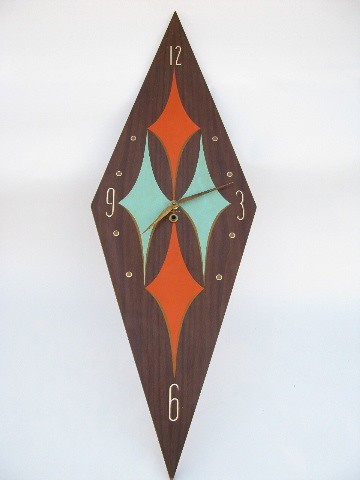This is a photograph of a diamond-shaped wall clock prominently displaying the numbers 12 at the top, 3 to the right, 6 at the bottom, and 9 to the left. The clock shows the time as approximately 7:12. The main body is crafted from dark brown wood, showcasing its natural wood grain. Behind the intricately designed gold hands, there is a pattern consisting of red diamond shapes at the top and bottom, with light aqua diamond shapes flanking either side. The clock is set against a light gray background, with noticeable shadowing towards the center of the paper upon which the clock rests, adding depth to the composition.